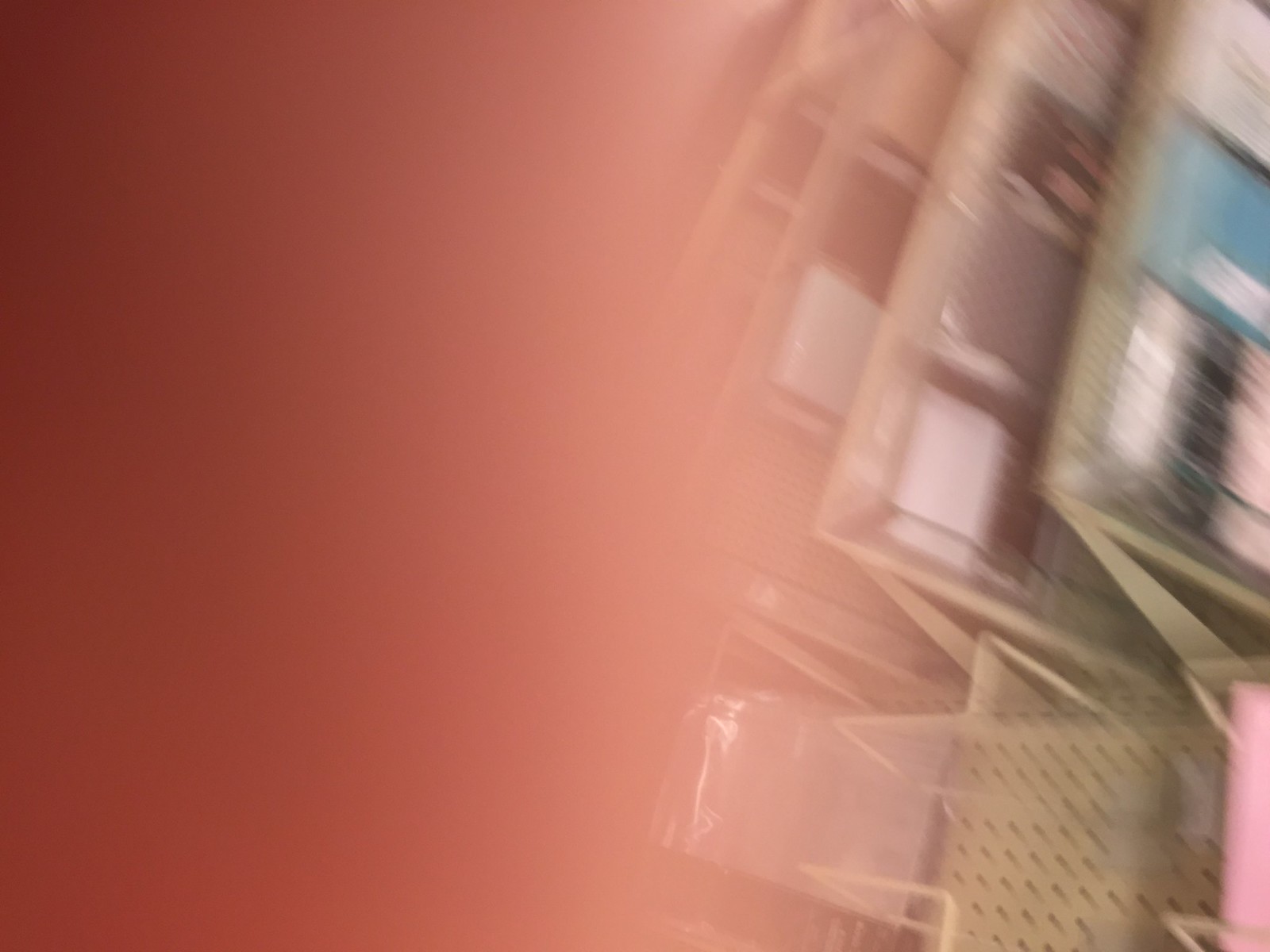This photograph is an extremely blurry image of store shelves. On the left side, the image is obscured by someone's finger, presenting a dark reddish-pink hue that fades as it transitions into the clearer part of the image. The right side reveals metal store shelves, likely yellowish-gray in color, arranged in an upside-down v-shaped pattern. The shelves are stocked with various stationary items, including notepads, planners, and journals. Specific visible items include a teal book, a white book, a black and white book with pink on it, and an entirely pink book located in the bottom right corner. The photograph appears to have been taken at an angle while the camera was moving, making it difficult to discern fine details. There are multiple shelves, and the objects on the lowest visible shelf, from left to right, include a blank space, a white item, a red item, and a pink item.